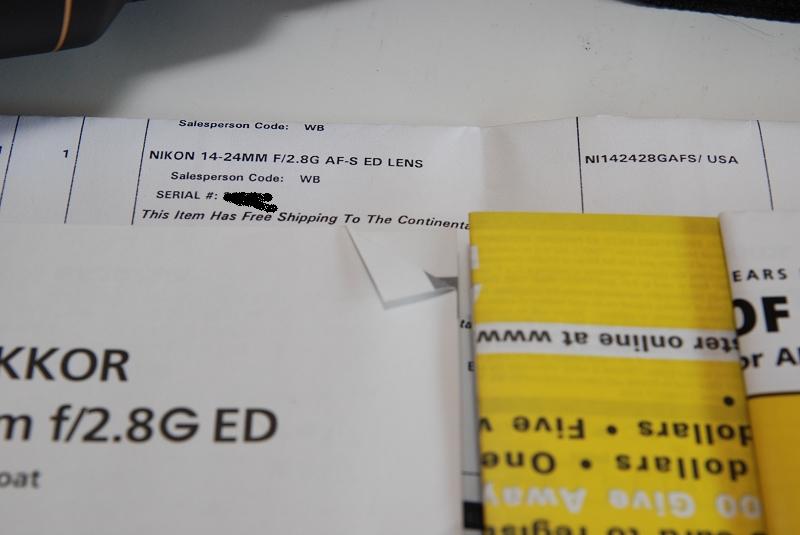This rectangular image captures the long side extending horizontally from left to right. The primary subject is a folded sales receipt for a Nikon lens, emphasizing the item **Nikon 14-24MM F/2.8G AF-S ED**. The readable portion includes details such as the salesperson code "WB", but the serial number is obscured in gray. The receipt mentions that this item comes with free continental shipping. However, part of the receipt is obscured by another piece of paper. Below this obscuring paper, there's a larger number, though the exact digits are not detailed in this description.

Additionally, several booklets rest atop the receipt. While these booklets are slightly out of focus, a white one with dark writing is discernible on the left. Another booklet on the right, characterized by both black and white writing on a yellow background, is notably upside down. This intricate composition provides a clear and comprehensive view of the essential elements related to a Nikon lens transaction, accompanied by some informational pamphlets.